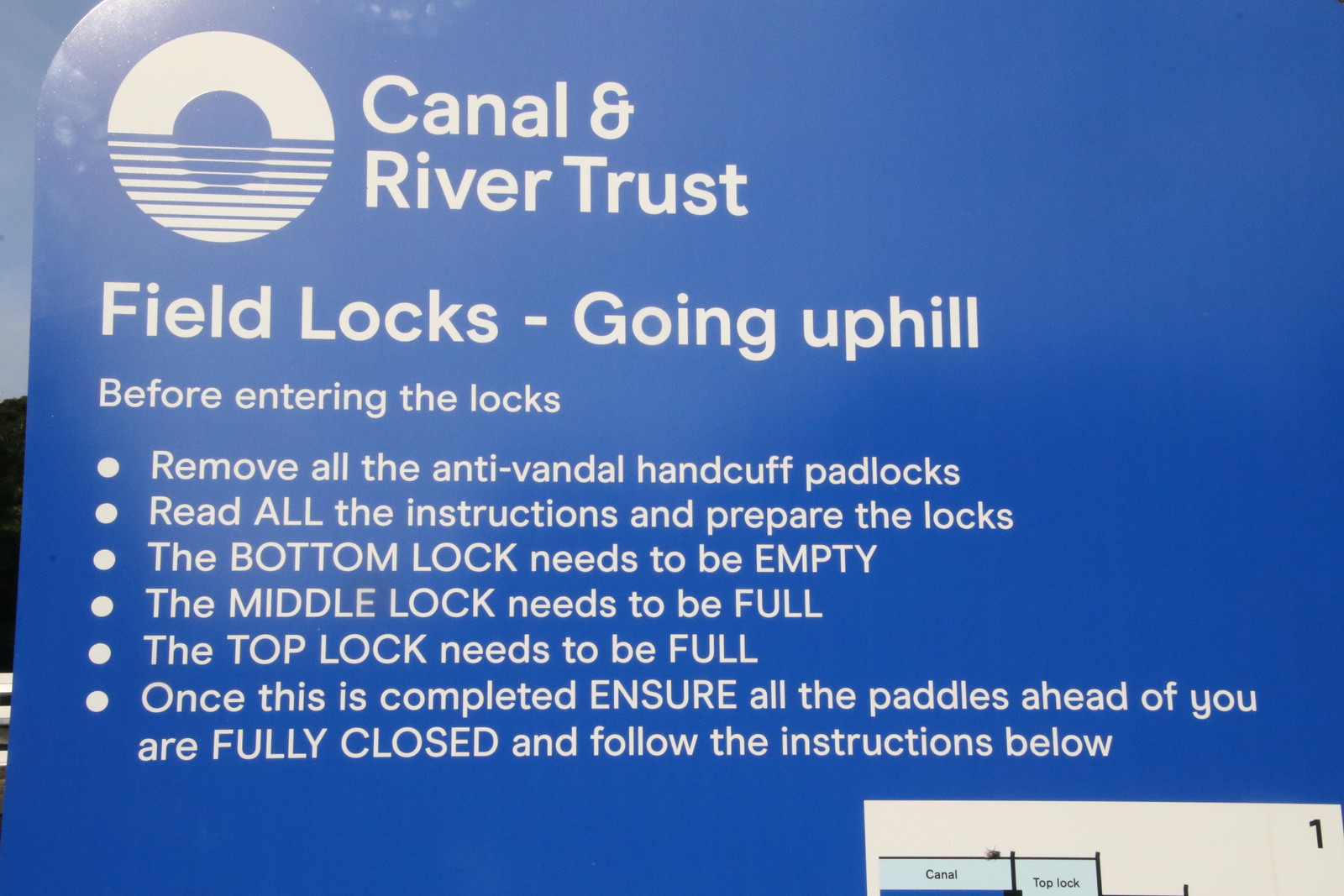The image is of a safety sign for a canal or river, specifically from the Canal and River Trust organization. The sign, predominantly blue with white text, provides detailed instructions for navigating “field locks going uphill.” Essential steps include removing all anti-vandal handcuff padlocks before entering the locks, thoroughly reading instructions, and preparing the locks according to specific requirements: the bottom lock must be empty, while both the middle and top locks need to be full. Once these steps are completed, ensure all paddles ahead are fully closed and proceed to follow further instructions. The sign’s text, where certain words are capitalized for emphasis, is predominantly centered, and a logo for the Canal and River Trust is displayed in the upper left corner. The overall style is a photograph, capturing the sign which fills the entire horizontal frame. The color scheme includes blue, white, black, and gray.